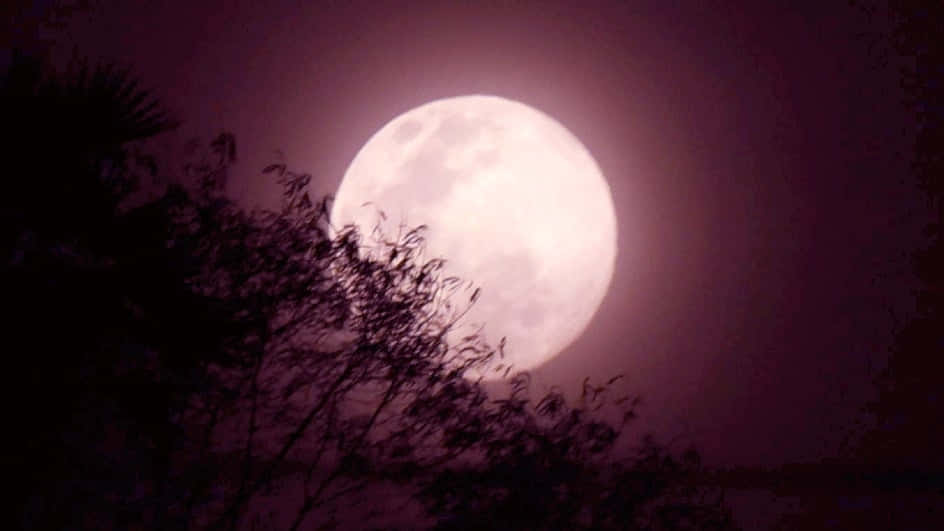The photograph captures a striking full moon set against the night sky. The moon, centrally positioned, radiates a bright white light tinged with hues of purple, maroon, and pale pink. Detailed textures and pitted shadows are visible on the moon’s surface, enhancing its celestial allure. Encircling the moon is a subtle halo, adding to its ethereal glow. In the foreground, the silhouetted branches of a tree, adorned with small oval-shaped leaves, provide an intricate contrast against the luminescent moon. These branches stretch diagonally from the top left to the bottom right of the image, partially obscuring the bottom left quadrant of the moon. The scene is enveloped in darkness, with the moon's radiant light fading into black at the corners, emphasizing the nocturnal ambiance. The slight motion in the tree hints at a gentle breeze, adding a dynamic element to the tranquil nightscape.